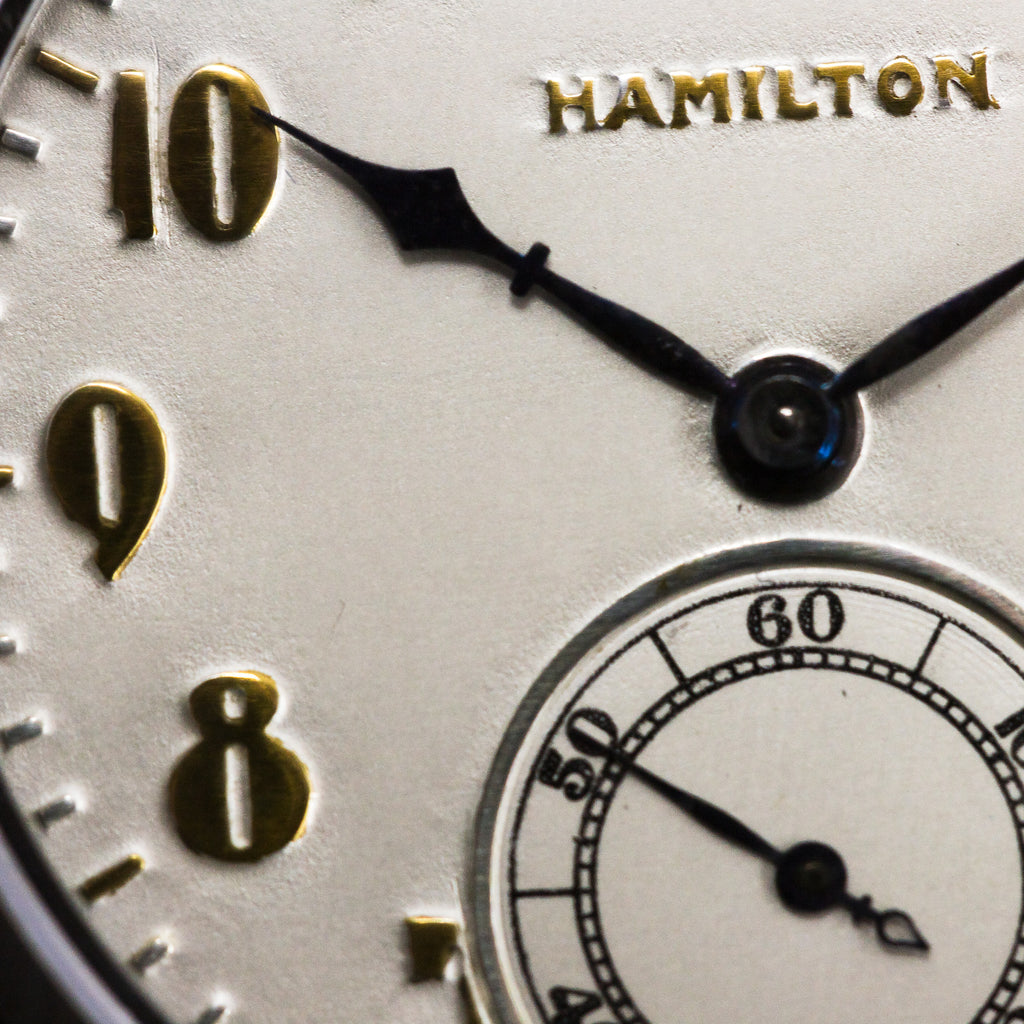This image captures a close-up of a sophisticated Hamilton clock face, predominantly featuring a white background. The partial clock face reveals the gold-painted numbers 10, 9, 8, and a part of 7, along with minute markers between them, also in gold. The brand name "Hamilton" is prominently placed in gold lettering above the central meeting point of the black hour and minute hands. The hour hand is positioned at 10, suggesting the minute hand is likely at the 2 o'clock mark, although out of frame. Below the main hands is a smaller, circular sub-dial with black numbering and hand, showing the seconds. In this sub-dial, the numbers 40, 50, and 60 are visible, with the second hand pointing directly at 50. The captured time appears to be approximately 10:20 and 55 seconds.